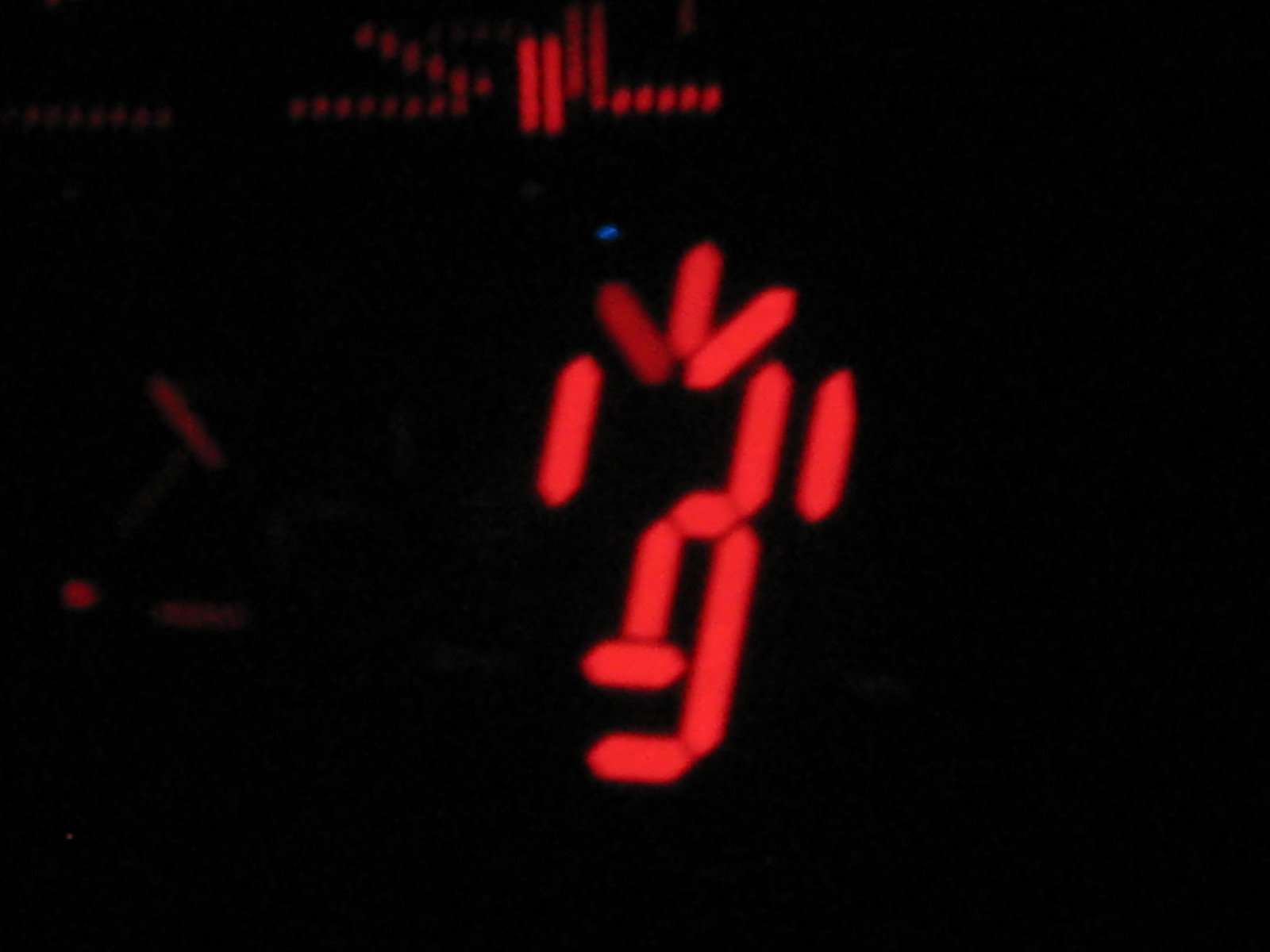The image depicts a dark, almost pitch-black background illuminated by red neon lines forming an abstract pattern. At the center, red lines, resembling a malfunctioning digital clock display or a glitched set of numbers, take prominence. These lines vary in orientation, with some vertical and others connected horizontally, creating an intricate, almost non-numerical arrangement. Interspersed are faint red dots and lines that spread across the scene, becoming more concentrated towards the middle and top sections. Adding to the complexity, there's a blue dot slightly below the center, surrounded by additional clusters of red dots and lines, some forming shapes reminiscent of a distorted figure or abstract symbol. The overall effect is a mysterious, dark canvas punctuated by these vibrant, chaotic red and blue elements.